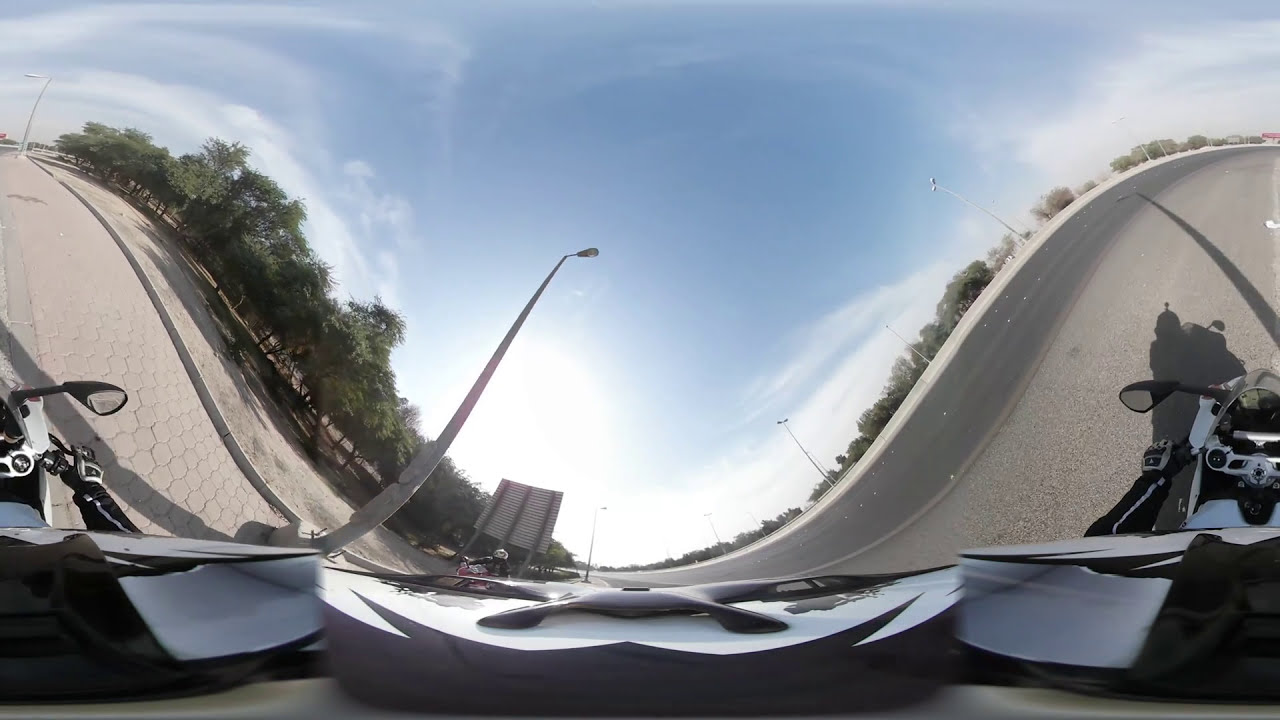This image is a highly distorted, almost 360-degree panorama view from the vantage point of a rider's helmet or a GoPro camera mounted on their head. The central subject is a motorcyclist wearing a black motorcycle jacket with silver stripes and black gloves. The picture depicts the rider on a road that appears to curve dramatically, creating a surreal wavy effect where the left side looks like it climbs steeply uphill and the right side descends sharply. The rider is near the edge of the road, close to a pentagon-shaped red brick sidewalk. The scene is illuminated by bright daylight with clear blue skies and soft clouds. Green trees and bushes are visible in the background along with some dividers and a street sign. Two streetlights are on either side of the road, and another motorcycle is seen further in the distance on the otherwise empty gray road. The image captures the solitude of the ride with very few other vehicles present.